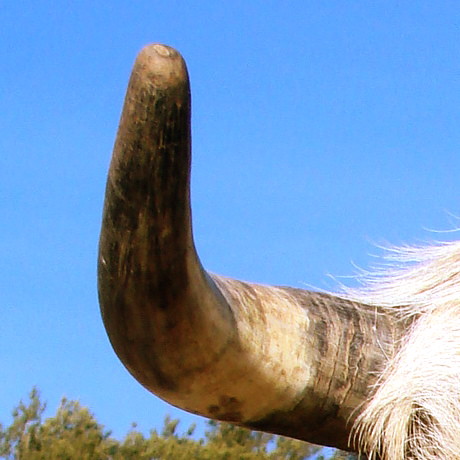The image shows a close-up of a large horn, presumably from a cow, extending prominently from the right side of the frame. The horn, which is not sharp but rounded at the tip, emerges from a patch of white, hairy fur at the base. Its texture appears weathered, displaying hues of brown that transition from a darker shade near the base to a lighter tan in the middle, with subtle streaks of darker brown further along. The horn curves to the left and upwards against a backdrop of a clear blue sky, with no clouds visible. At the very bottom of the image, the tops of green trees can be seen, adding contrast to the otherwise serene blue background.